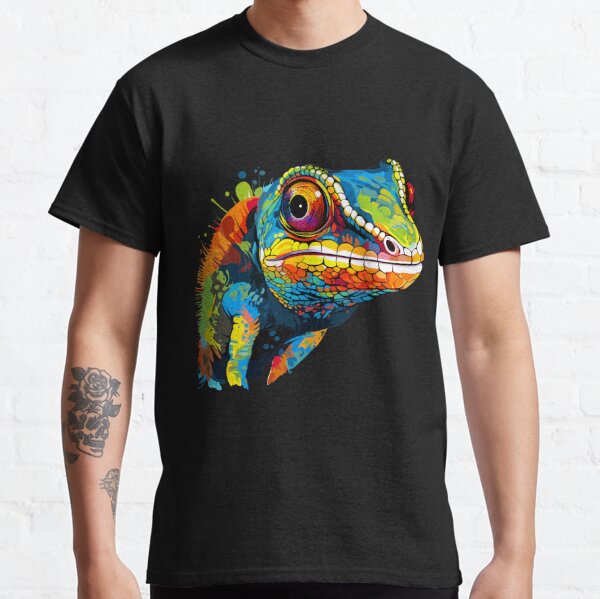The image features a model showcasing a black, round-collar t-shirt against a white brick wall. The model, who appears to be Caucasian, is shown from the neck down, and a distinct tattoo of a skull with flowers emerging from it adorns their right forearm. The t-shirt prominently displays a colorful screen-printed image of a lizard with a side profile view of its face and feet. This eye-catching reptile design is detailed with vibrant colors, including shades of red, orange, yellow, green, blue, purple, and white, particularly highlighting its ridge-like crown and human-like teeth. The model's lighter skin tone and the clarity of the image are enhanced by natural lighting, making the details of both the tattoo and the t-shirt's artistic reptile graphic stand out vividly.